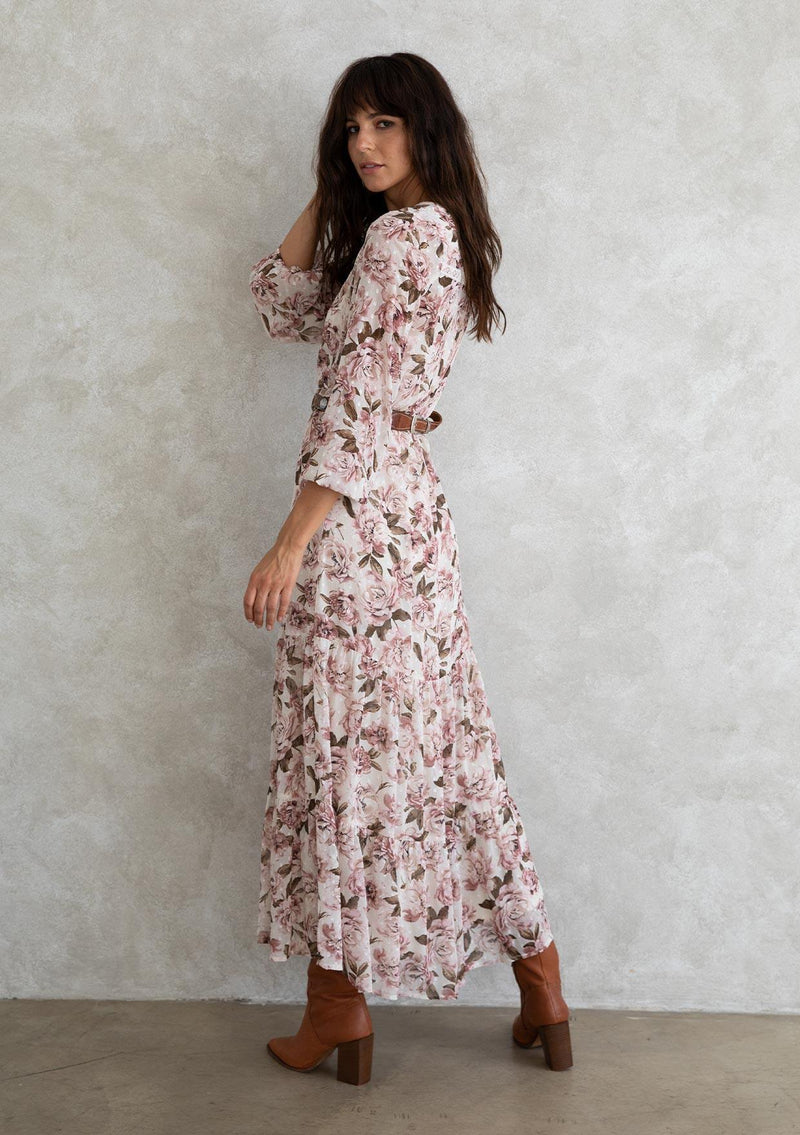The image depicts a beautiful white woman, modeling in front of a white wall with a grayish stone-like texture. She is standing with her legs slightly apart on a light brown floor. She is wearing a long, elegant, pink and white floral dress that reaches down to her ankles. The floral patterns on the dress feature darker shades, like brown or black. The dress is cinched at the waist with a tan belt. She has long dark brown hair styled with bangs and is wearing light brown, short-heeled, leather boots. The woman strikes a provocative pose, looking over her left shoulder towards the camera with her right hand reaching up towards her hair on the right side of her head.